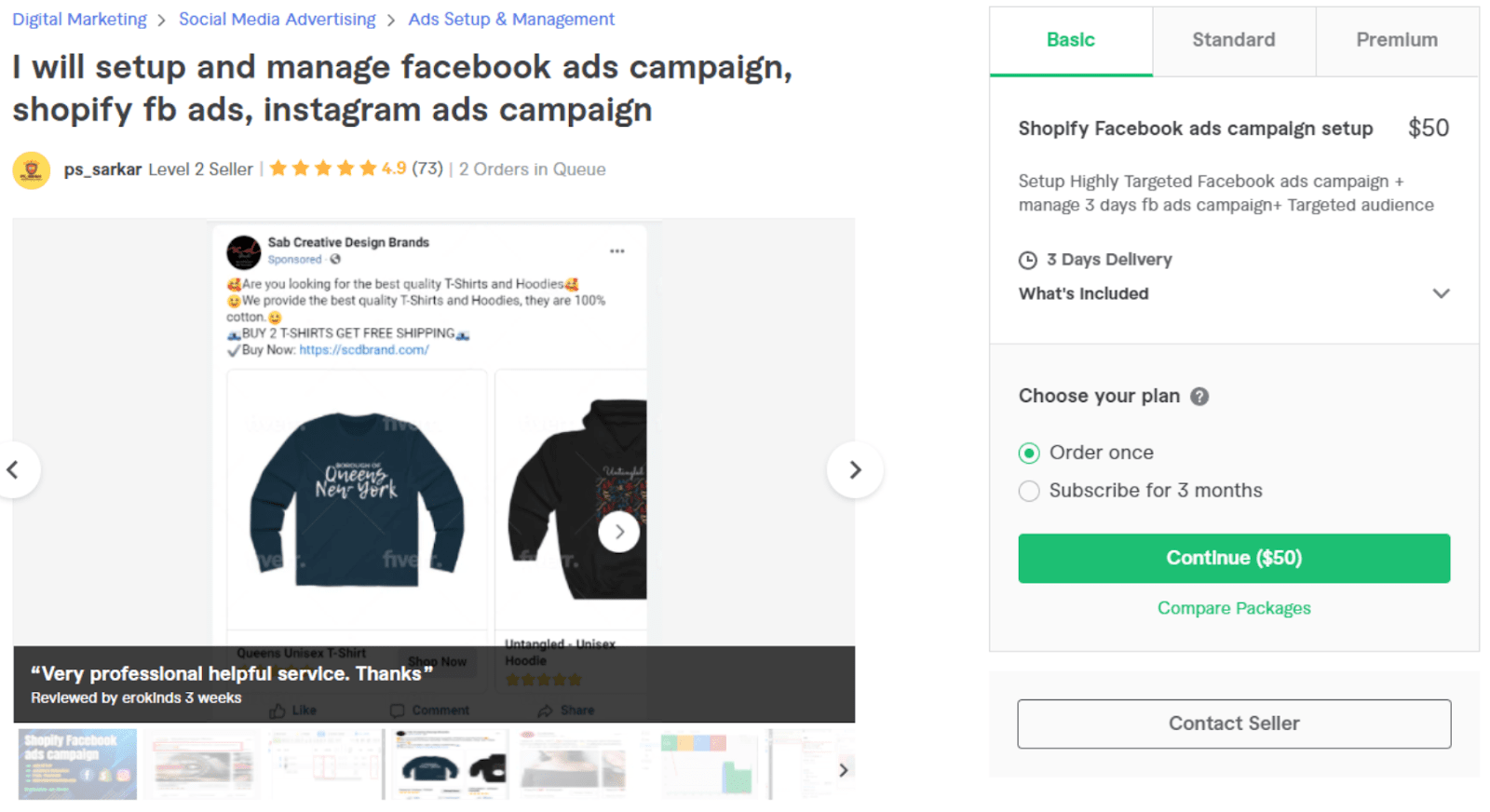**Descriptive Caption:**

This is a screenshot of a desktop or laptop computer displaying a web store that offers various digital marketing services, particularly focused on social media advertising, ad setup, and management. The platform resembles popular freelance marketplaces like Fiverr, where users can sell their specialized services to others.

The featured service highlights the expertise in setting up and managing Facebook and Instagram ad campaigns, as well as Shopify FB ads. The listing is titled "I will set up and manage Facebook ad campaigns, Shopify FB ads, Instagram ad campaigns," emphasizing a professional and helpful service. 

Reviewed by user Erokind three weeks ago, the ad includes a sample image showcasing previous work. The service provider, PS Sarkar, is a Level 2 seller with an impressive rating of 4.9 stars from 73 reviews and currently has two orders in queue. 

On the right side of the page, there are three service tiers available: Basic, Standard, and Premium. The Basic plan, which is selected, costs $50 and includes the setup of a highly targeted Facebook ads campaign, management of the campaigns for three days, and targeted audience selection. Delivery for this service takes three days. 

Potential customers can choose to order once or subscribe for three months. Below this, there's an option to continue with the $50 Basic plan or compare it with other packages. Additionally, there's a "Contact Seller" button for direct inquiries.